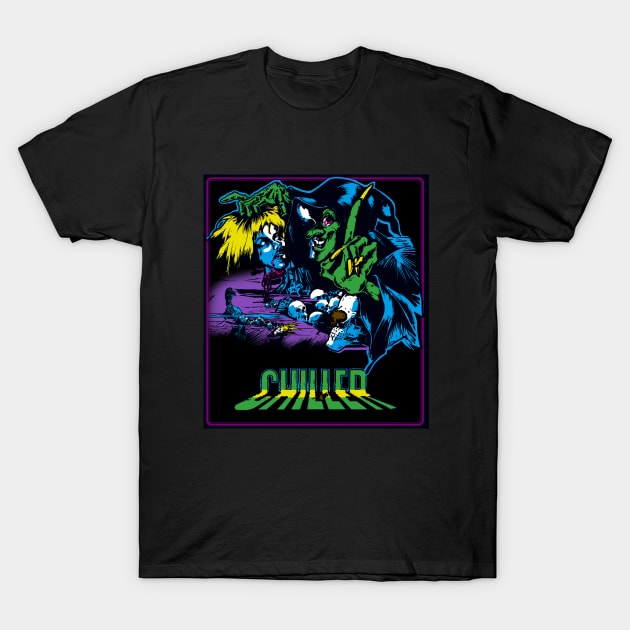This is an image of a black, short-sleeve t-shirt laid flat against a neutral off-white background. The t-shirt features a centrally placed graphic design, bordered by a bold purple outline. Within this purple-bordered box is a dynamic and dark scene, drawn in a pixel art style with a predominantly black background. The scene includes a green-skinned character, resembling a witch or goblin, with long green fingers tipped with pointed yellow nails. This character is depicted holding up one finger, and its face is green with black hair and a bloodshot eye. Below this central figure, there are multiple skulls and possibly metal tools scattered around. To the left of the green-skinned character is a dismembered head of a blue-faced figure with yellow hair. The base of this eerie scene seems to float on a purple island within a black void. At the bottom of the graphic, the word "Chiller" is prominently displayed in green letters, intersected by a yellow stripe that distorts the text slightly. Overall, the t-shirt's design conveys a chilling, cartoonish, and somewhat surreal aesthetic.